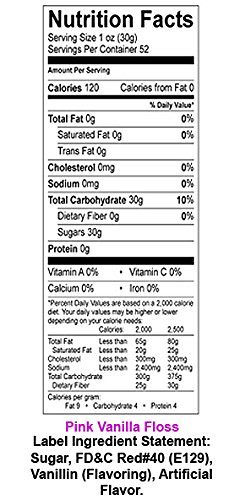This image shows a detailed Nutrition Facts label, which is long and rectangular in portrait orientation. At the top, it reads "Nutrition Facts," followed by information on serving size and servings per container: one ounce (30 grams) per serving, with a total of 52 servings per container. Below this is a bold horizontal line and the phrase "Amount Per Serving" in a small font, followed by "Calories 120," and "Calories from Fat 0."

The label continues with the percentages of the daily values and lists the following nutrients: total fat 0 grams, saturated fat 0 grams, trans fat 0 grams, cholesterol 0 milligrams, sodium 0 milligrams, total carbohydrate 30 grams, dietary fiber 0 grams, sugars 30 grams, and protein 0 grams. Another bold horizontal line separates this section from the subsequent information.

At the bottom of the Nutrition Facts label, additional product information is provided: "Pink Vanilla Floss," followed by "Label Ingredient Statement." The listed ingredients include sugar, FD&C Red #40 (E129), vanillin, and artificial flavoring. This nutrition label resembles a standard United States label, despite the uncertainty about the food item's origin. The nutritional content indicates it is not a particularly healthy option, given its high sugar content without other nutritional benefits.